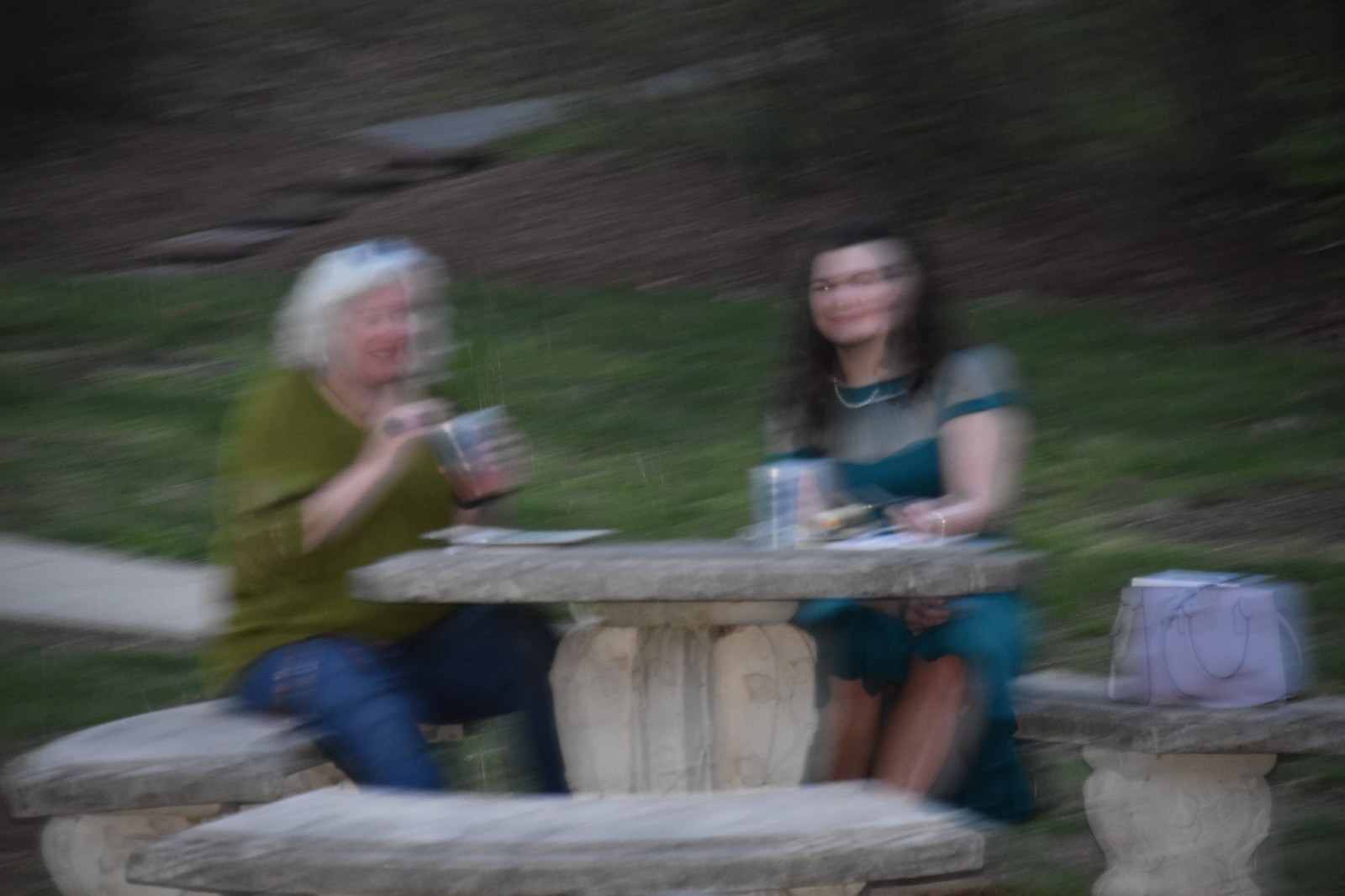In this very blurry color photo, two women are sitting at a circular stone table in a park. The image appears smeared, likely due to camera movement, giving a double-exposure effect to their faces and surroundings. The table is a gray, round pedestal type with three curved stone benches around it. On the left sits an older woman with white shoulder-length hair and sunglasses propped on her head. She’s wearing a green short-sleeved top and blue jeans, her sleeves rolled up. She is holding up a cup or container in her left hand, with her right hand hovering above it. To her right is a younger woman with long, dark hair wearing a short-sleeved, cap-sleeved, teal dress. A lavender-colored handbag rests on the bench beside her and she has a cup in front of her on the table. Both women appear to be smiling as they eat, although their faces are distorted by the blur. The background includes some grass, shallow steps, and a pathway leading into an area with landscaping and brown mulch.